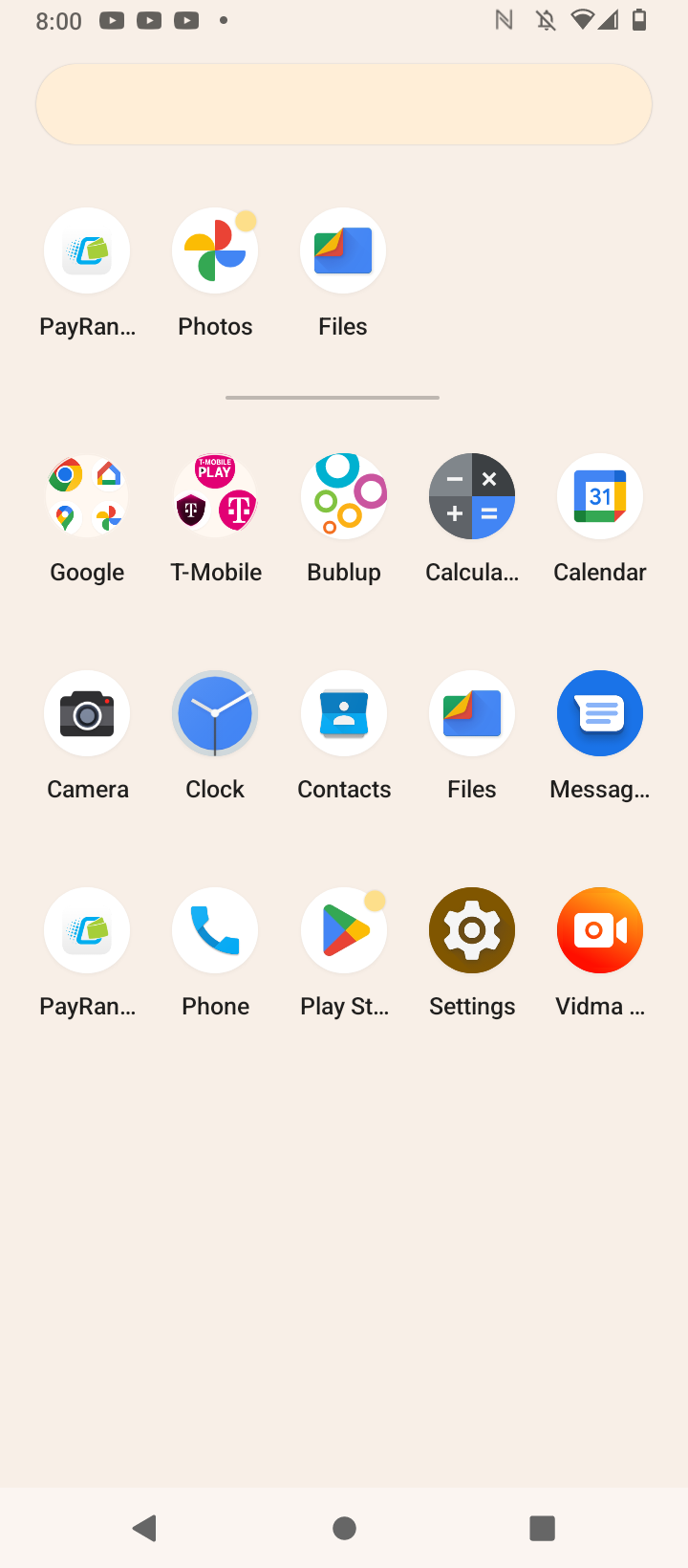The screenshot captures a cell phone screen at precisely 8:00. The status bar at the top shows a Wi-Fi symbol and a battery icon indicating approximately 50% charge. The primary display features various app icons, each distinct and easily recognizable. 

Prominently, there are three play buttons visible. The T-Mobile logo, in shades of pink and white, also reads "play." The Google Drive app icon is characterized by its triangular logo in blue, red, yellow, and green. Nearby, is the calculator icon displaying arithmetic symbols (plus, minus, equal, and multiplier signs) for quick mathematical access.

Additionally, there is a calendar icon marked with the number "31," a camera icon, and a clock icon. The screen includes app shortcuts for Contacts, Files, Messaging, and a Phone app represented by a white icon featuring a blue telephone handset. Lastly, a cog-shaped Settings icon is also present, providing quick access to the phone's configuration options.